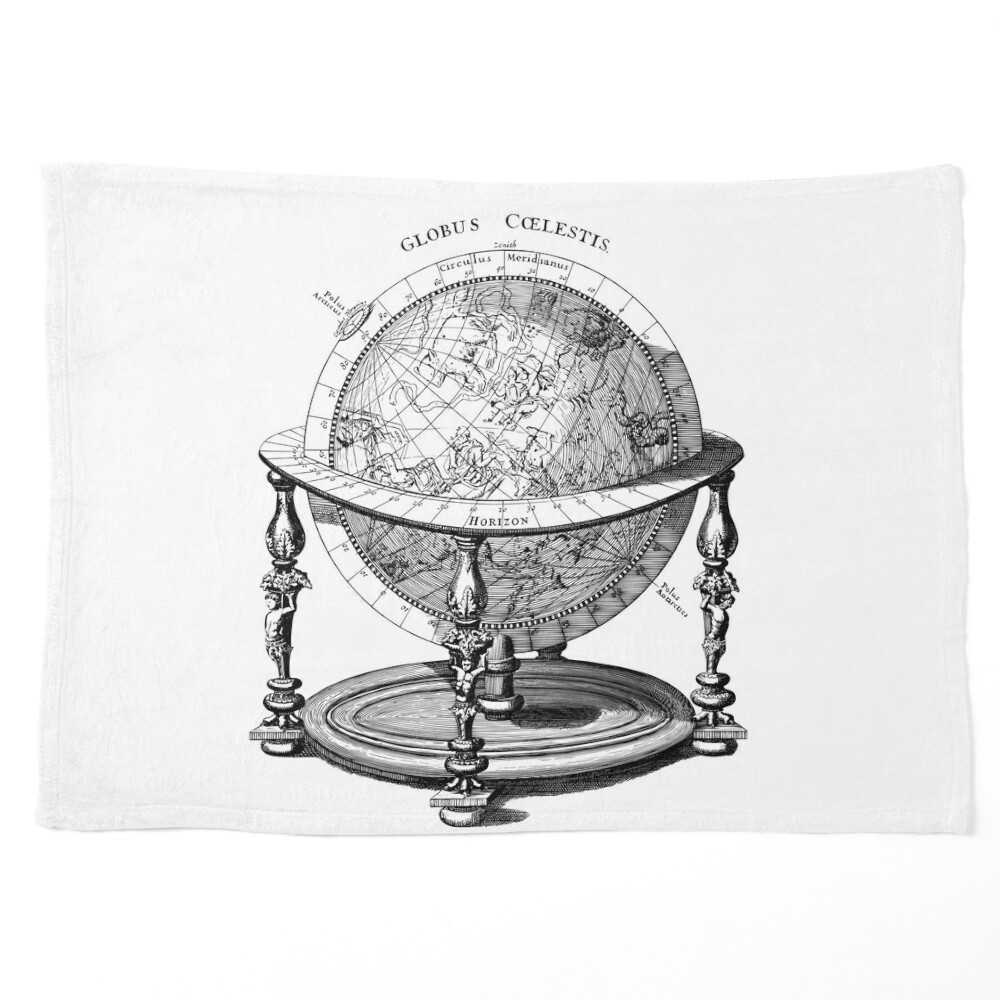The image features a highly detailed, grayscale hand-drawn globe referred to as "Globus Celestis" in small text above it. This celestial globe showcases constellations rather than geographical outlines, with intricate sketch-like lines to depict various astronomical elements. The globe is supported by an ornate and unique holder consisting of three slim, wooden posts shaped like men without shirts, tied to the posts, each holding flowers. These figures support the globe, which sits on a gray plate. Encircling the globe are various numbers that mark longitude and latitude, aiding in celestial navigation. The structure horizontally bisecting the globe is labeled "horizon" and "circulus meridianus," delineating significant celestial markers. At the top of the globe, another label reads "Holus Academus," adding to the intricate detailing that defines the image.